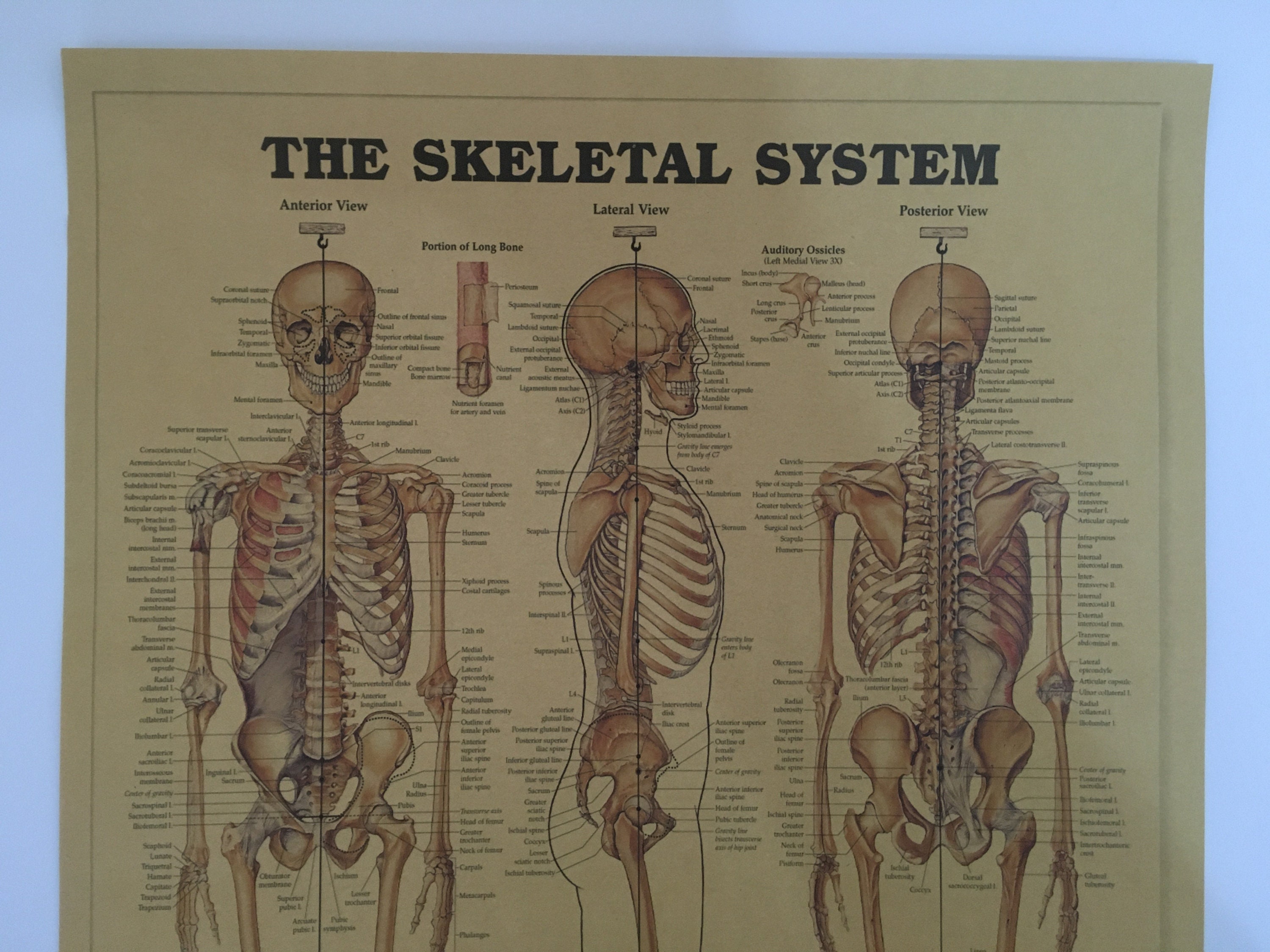This image is a detailed photograph of an educational poster titled "The Skeletal System," prominently written in black block letters at the top. The poster, set against a black background, features three detailed images of a skeleton: an anterior view (front), a lateral view (side), and a posterior view (rear). Each skeleton illustration, in light brown hues with accompanying small black text, meticulously labels every bone and visible structure.

Between the heads of these skeletons, there are small inset graphics highlighting specific parts of the body. The background of the poster is a neutral tan or grayish beige, providing a clear contrast to the black text and labeled structures that make up the skeletons. This poster, designed for educational environments such as anatomy classes or doctor's offices, includes small, intricate graphics that provide enlarged views of selected bones for greater detail. Though it's challenging to discern gender from the imagery, the poster remains a comprehensive visual aid for studying the skeletal system.